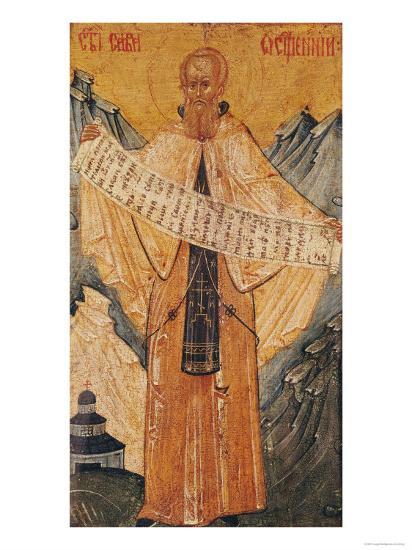The image appears to be an aged, rectangular illustration from a book, aligned vertically. It depicts an older man with short, receding hair and a long, orangey-blonde beard. His face, colored in a brownish hue, shows a prominent forehead and a narrow jaw, giving it an upside-down jug-like shape. 

The man is adorned in a large, brown robe with a whitish-brown cape draped over his shoulders. A narrow black strip, embellished with a cross, hangs from his neck down to his legs. Holding a long white scroll with indistinguishable brown scribbles, the man's arms are extended outward, creating a diagonal slant, with his left arm positioned higher than his right.

The background is a blend of brown tones, with blackish mountains flanking him on either side. Red lettering in an ancient, unreadable script occupies the top left and top right corners of the image. The lower left corner features a small, circular dome building, while the lower right corner displays a pattern resembling jagged rocks or a feather. The perspective throughout the illustration appears skewed, further emphasizing its old and weathered appearance.